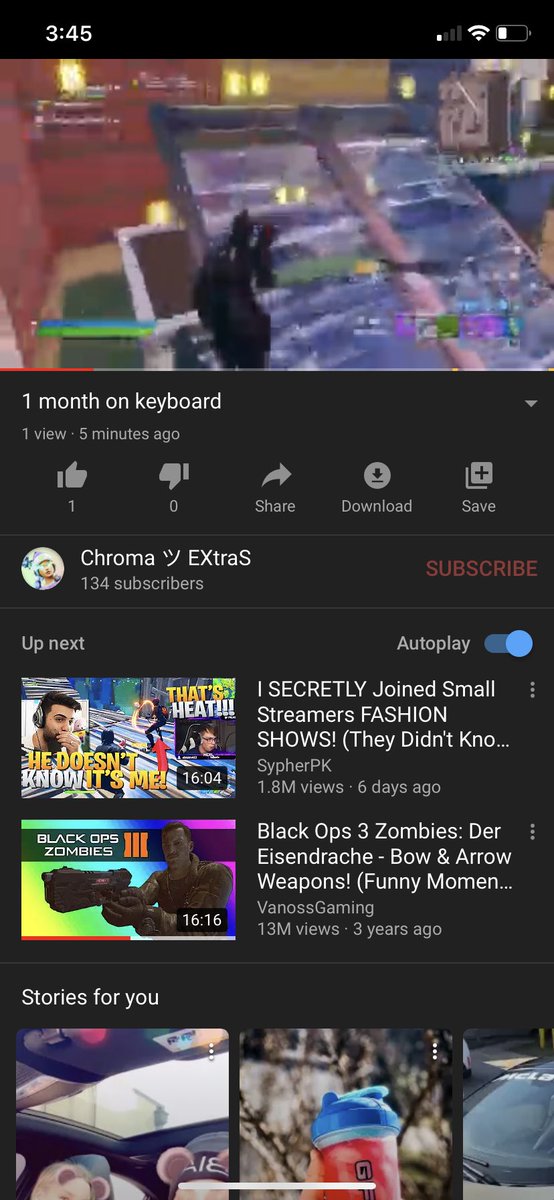A screenshot depicts a phone app, potentially YouTube or Twitch, showcasing a video interface. At the top of the screenshot, a blurred and blocky image of someone playing what appears to be Fortnite is visible. The video's progress bar, colored red, indicates that around 15% of the video has been played.

Underneath the video, text reads "one month on keyboard." Additional video details are shown, such as "one view," "five minutes ago," and engagement icons for a thumbs up (one) and a thumb down (zero), as well as options to share, download, and save the video. The video's creator is identified as Chroma Extra, with ‘EX’ and 'S' in "Extra" capitalized, and has 134 subscribers. The creator's profile image features their face with sunglasses and a cap, along with a small logo.

To the right of this section is a "SUBSCRIBE" button. Below, there are two video thumbnails. The first is titled "He Doesn't Know It's Me: I Secretly Joined Small Streamers' Fashion Shows They Didn't Know" by CypherPK, with 1.8 million views in six days. The second video, titled "Black Ops Zombies," runs for 16 minutes and 16 seconds, while the first is 16 minutes and 14 seconds. Additional text in German is visible under the "Black Ops Zombies" title, referencing "Bow and Arrow Weapons, Funny Moments" by VanossGaming, which has garnered 13 million views over three years.

At the bottom of the screenshot, there are various photographs, including G Fuel advertisements and unclear images that appear to be taken inside a car.